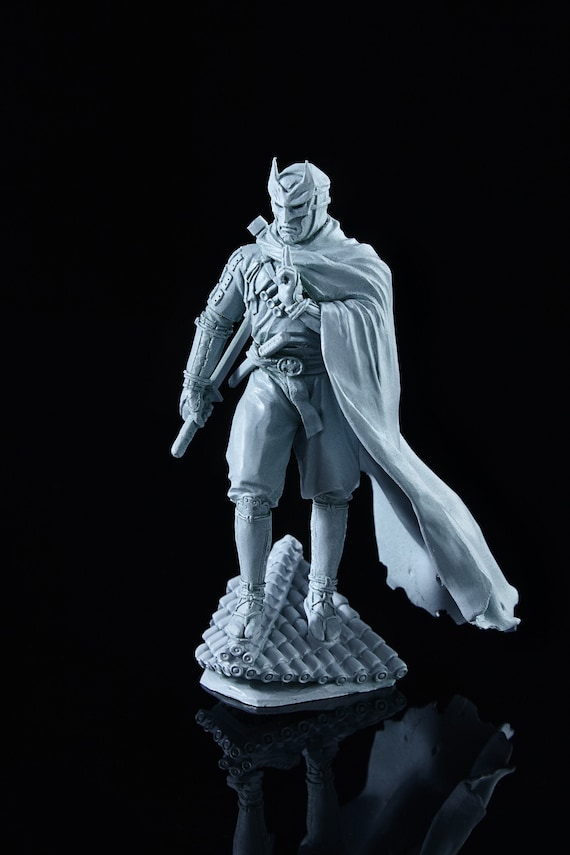This image features a detailed miniature statuette of an enigmatic superhero or warrior figure, posed against a stark black background. The statuette is cast in a bluish-white material that resembles marble, and the glossy black surface it stands on creates reflective interplay highlighting the intricacies of the figure. Wearing a mask that wraps over his face and sports pointed, ear-like protrusions akin to a bat cowl, the figure exudes an old-fashioned yet heroic aura. His long, flowing cape drapes dramatically over his right shoulder, sculpted with such precision that it mimics the texture of real fabric.

The miniature is dressed in a shirt with decorative buttons on the shoulders, blousy knee-length pants, knee-high socks, and open-toed rope sandals. The protagonist's feet reveal sandals held in place by thongs that slide between his toes. A robust sash with a prominent buckle cinches his waist, and attached to it is a sword resting against his hip, ready for a swift draw. Additionally, he holds a long staff-like object with one hand, perhaps a weapon like a hammer or another sword, though its features remain ambiguous. The confident and fierce expression on his face is captured as he gazes downward, imparting a sense of vigilance.

The hero's pedestal is a small, tiled rooftop segment, hinting at a vigilant stance atop a building. The figurine's high level of detail suggests it could be part of a larger narrative world, possibly from a chess set or as a standalone collectible.